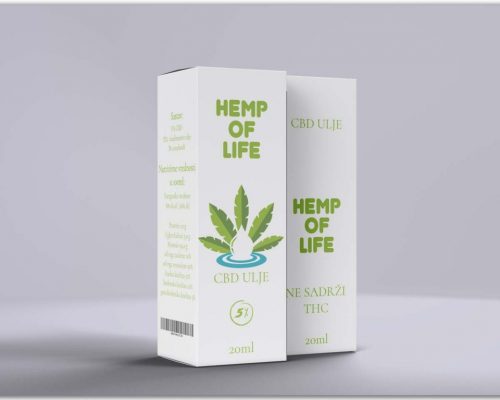The image is a color photograph in landscape orientation featuring two tall boxes against a grayish-white background, with shadows cast underneath them. The boxes appear to be a product called "Hemp of Life," which is a CBD supplement. The box on the left displays a dark green font with the text "Hemp of Life" at the top, followed by an illustration of a hemp leaf encircling a white droplet in a blue pool, symbolizing purity and perhaps the liquid form of the product. Below this illustration, the text reads "CBD ULJE," "5%" within a circle, and "20 ml" at the bottom. This box also has additional text and a UPC code on its side, partially visible yet too light to fully discern. The box on the right mirrors the text of the left box but lacks the hemp leaf illustration, displaying only "CBD ULJE," "Hemp of Life," "5%," and "20 ml." The light gray background subtly suggests a curved tabletop where the boxes are placed, enhancing the realism and representational style of the product photography.